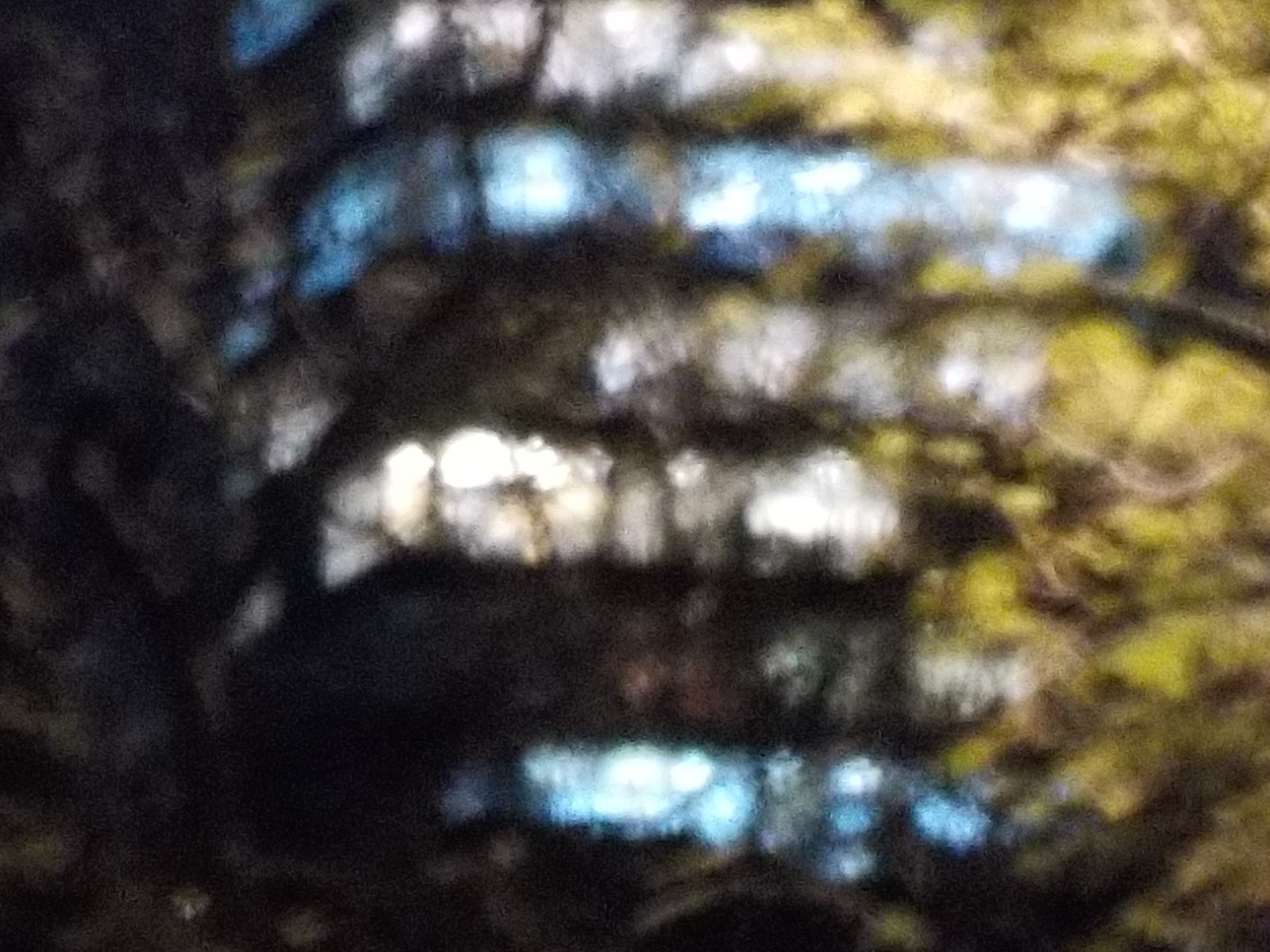The image is a very blurry nighttime photograph dominated by dark tones, giving an impression of an obscure, indistinct scene. The foreground is filled with numerous branches and leaves, more densely distributed on the left side than on the right. On the right side, some of the foliage is illuminated by an unidentified light source, highlighting green leaves among the branches.

In the background, a building can be discerned through the lines of branches. The building's facade features horizontal rows of neon lights in varying colors—blue and white—indicating different floors or sections. The top row displays blue lights, followed by white, alternating between the two colors, with multiple white-lit sections towards the middle and further blue lights at the bottom.

Although greatly out of focus, creating a predominantly brownish blur interspersed with green and blue hues, the image suggests a scene of an office block with its lights turned on at night, partially obscured by tree branches in the foreground.